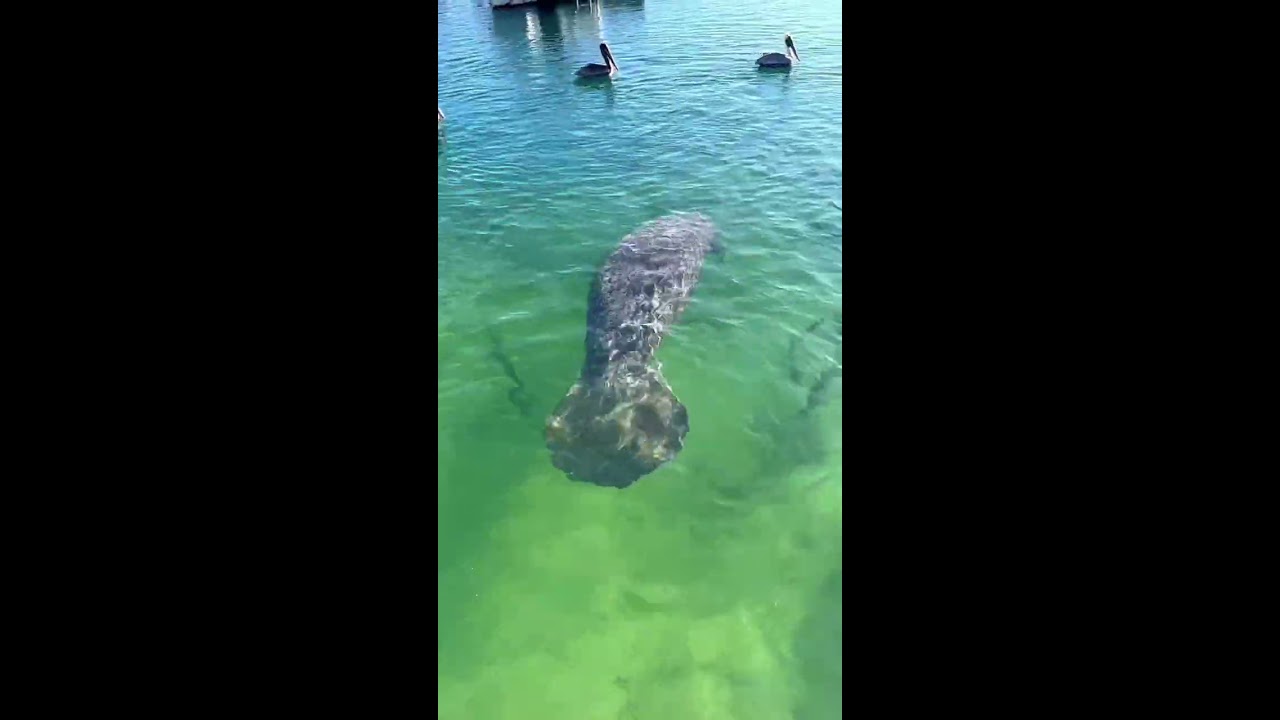The image features a body of water, likely a lake or a pond, with greenish-blue hues and gentle ripples suggesting a windy day. In the foreground, partially submerged, is a large gray animal, speculated to be an underwater creature such as a manatee, seal, or perhaps a beaver. The creature is positioned face down, making it difficult to identify conclusively. Two pelicans (or similar large water birds) swim in the background, adding a touch of wildlife to the scene. The image also hints at plant life beneath the water's surface. On either side of the color photograph are thick black borders, with no additional text or information. The overall composition suggests an outdoor setting captured possibly from a boat, evoking a sense of mystery around the unidentified aquatic creature.